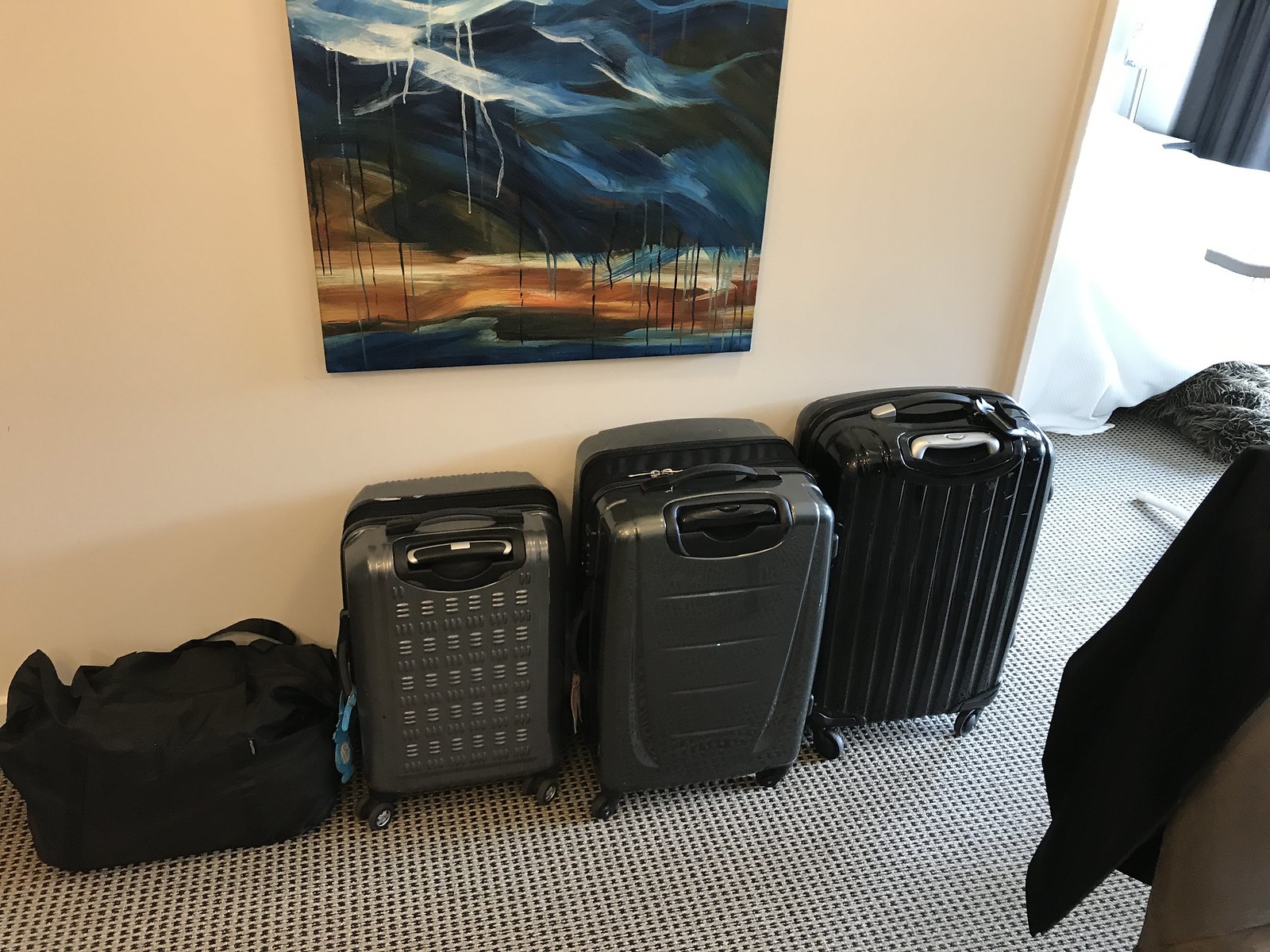The photograph depicts a hotel room characterized by its sparse, utilitarian design. Lined up against a beige tan wall are four pieces of luggage. On the far left is a black duffel bag, followed by a small grey and black hard-shell suitcase. Next to it is a larger, bulkier grey and black hard-shell suitcase, and on the far right is another black hard-shell suitcase. The floor is covered with a soft, small-checked carpet in brownish tones, adding a touch of subtle pattern to the room. A piece of abstract art, featuring swirls of blue, white, brown, and black, hangs on the wall above the luggage. To the right of the luggage, a portion of a bed with billowy white sheets is visible, along with some black curtains. Just peeking into the frame on the right side are what appear to be items of clothing, possibly jackets, further emphasizing the transient, lived-in quality of the space.